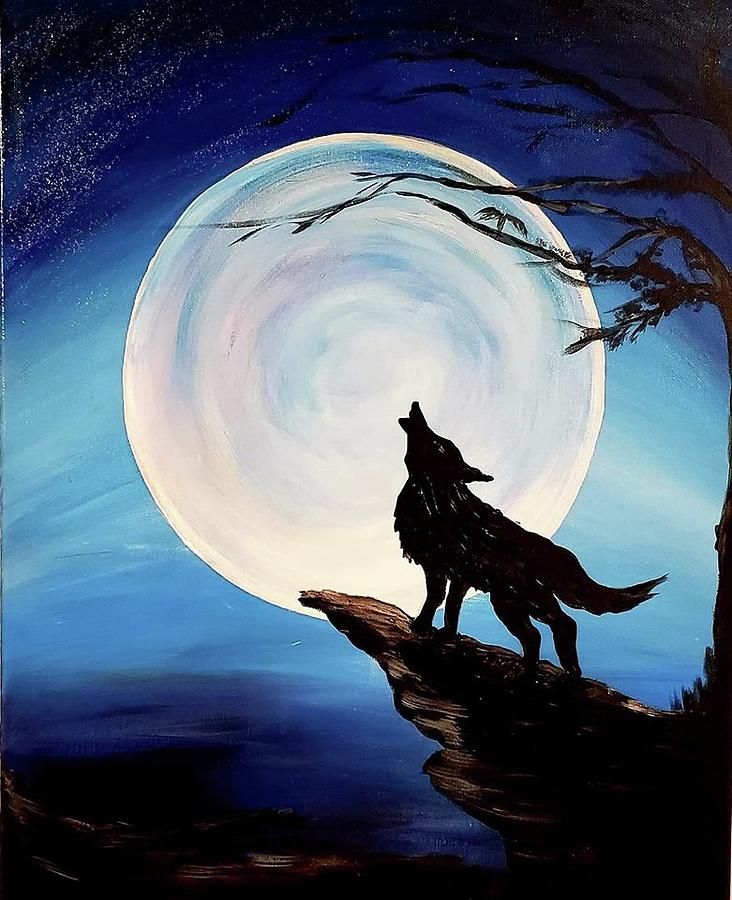This impressionistic and slightly abstract painting captures a mesmerizing night scene dominated by a massive moon that occupies nearly half the frame, adorned with hints of blue, purple, pink, and white. The night sky surrounding the moon is painted in a blend of streaky light blues and dark blues, dotted with numerous stars, particularly concentrated in the top left corner. A prominent black wolf, silhouetted in shadow, is positioned on a rock outcropping or crag in the bottom right of the composition. The wolf's body extends partly into the foreground of the moon, enhancing the depth of the scene. Additionally, a dark, shadowy tree with branches extends over the wolf and intersects with the moon, framing the focal point of the painting. The overall color palette is a harmonious blend of dark and light blues, blacks, and subtle starry accents, which together create a captivating nocturnal landscape.